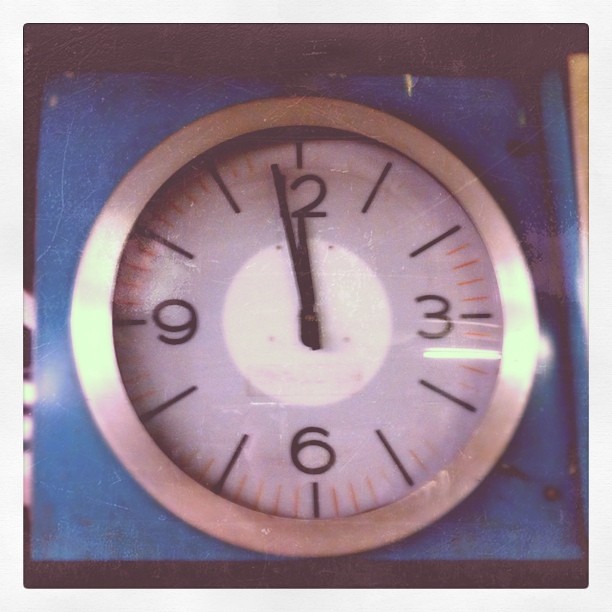This indoor digital photograph is primarily dark, featuring a consistent black background in both the upper and lower sections. On the left side of the image, roughly three-quarters down, an indistinct white object appears in the background. Near the upper right area is an element of light tan color. Dominating the right side of the picture is a blue square mottled with black specks. Within this square sits a striking silver clock encased in clear glass. The clock's face is a bright white, with a dazzlingly intense white circle at its center. It displays Roman numerals at the positions of 12, 3, and 6, all marked in black, while the other positions are denoted by large black lines. The black clock hands are set to 11:59, and there might be a second hand, potentially indicating 59 seconds, though it's indistinct and not clearly visible.